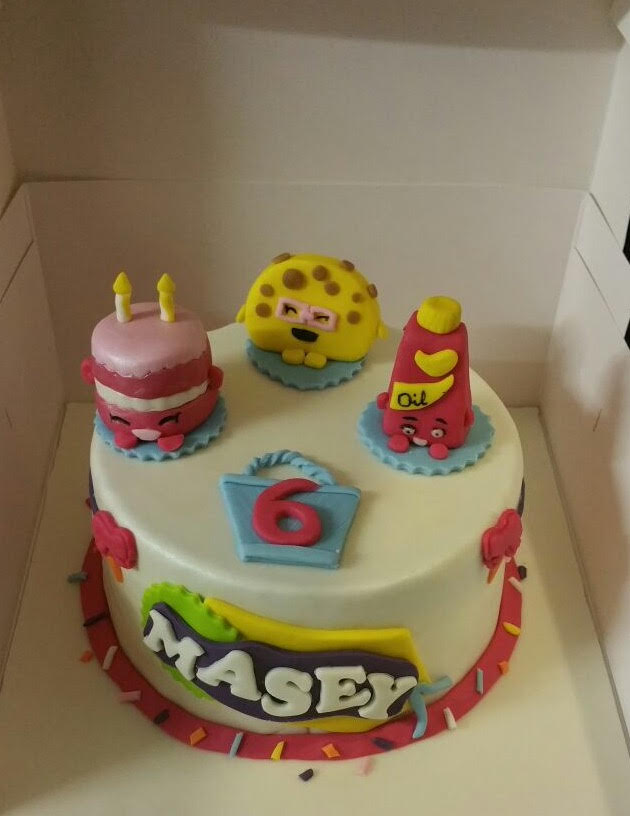The photograph showcases a detailed and whimsically decorated children's birthday cake inside an open white cardboard cake box. The cake, predominantly white with a red base, is festooned with colorful decorations in light blue, yellow, orange, and white. The front of the cake prominently displays the name "Macy," outlined with a green, purple, and yellow border. A unique fondant flower pot with a pink number six signifies Macy's sixth birthday. Whimsical, three-dimensional decorations heighten the cake's charm. These include a smiling pink miniature cake with two candles, a light blue basket shape with a red number six, a red bottle with a yellow cap labeled "oil," and a yellow taco-like creature donning pink glasses and brown spots. Each figure sits on a light blue frosting disc, adding to the playful and imaginative theme of the cake.